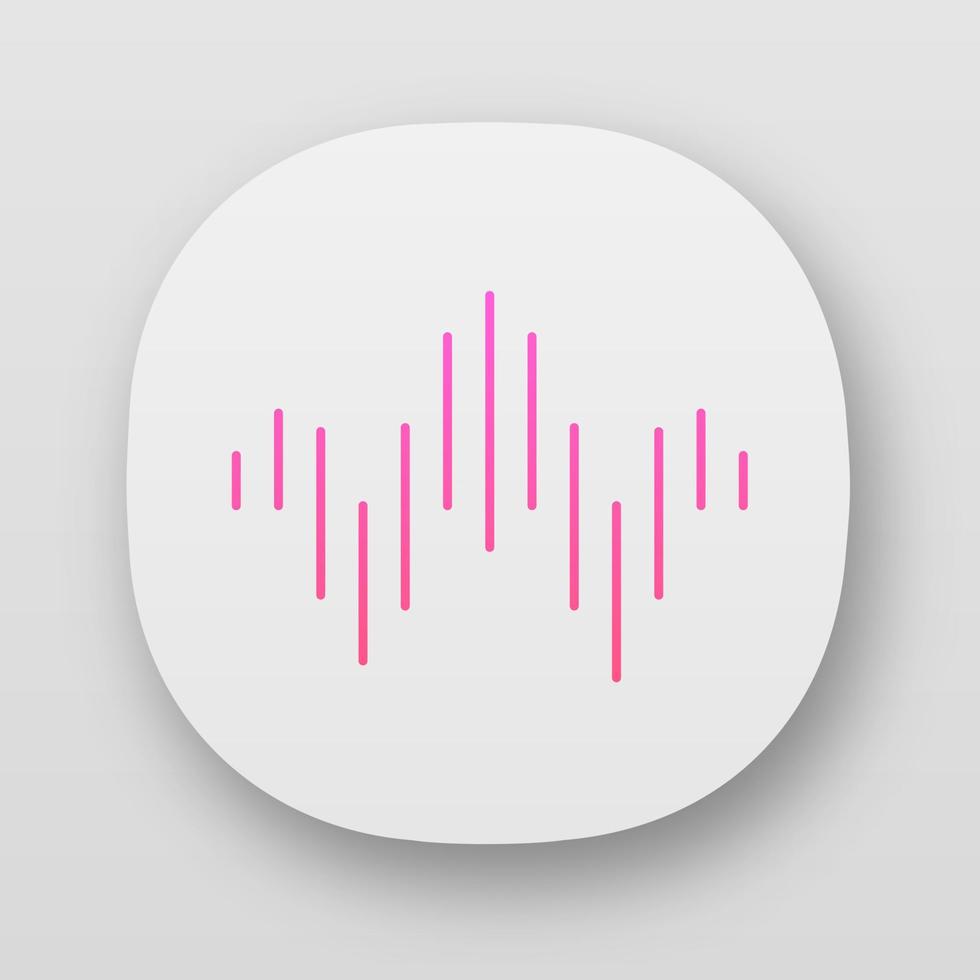This image features a white, square-shaped object with rounded corners set against a gray background. In the center of the square is a waveform pattern created by vertical lines. These lines vary in length, creating a visual effect that resembles a fluctuating graph or sound wave, dipping down and rising up sequentially. The lines exhibit a gradient coloration, transitioning from purple at the top to pink at the bottom. Behind the waveform, a white circle casts a subtle shadow, enhancing the three-dimensional appearance of the design. This object appears reminiscent of a charging pad for smartphones.